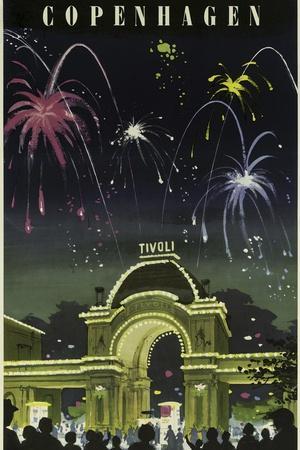This is an aligned rectangular, computer-generated image in portrait orientation, resembling a poster. At the top, "Copenhagen" is prominently displayed in a pale yellow, cream-colored, serif font, in all caps against a black sky. Below this, a grand architectural structure with a large arched center, topped with a dome and the word "Tivoli" inscribed at the top, dominates the middle of the image. This building appears to be stone brown, illuminated with yellow and green-gray tones. Surrounding the structure, the sky transitions from black at the top to a brownish gray towards the middle, filled with vibrant fireworks—dark pink on the left, white on the right, and light green above, each with swirled lines depicting their explosive trails. Silhouettes of a crowd, shaded in black, gather at the bottom of the image, while outlines of tree branches and leaves on the right frame the sides. This illustration captures a festive nighttime scene with meticulous detail and playful use of colors to evoke the lively atmosphere.